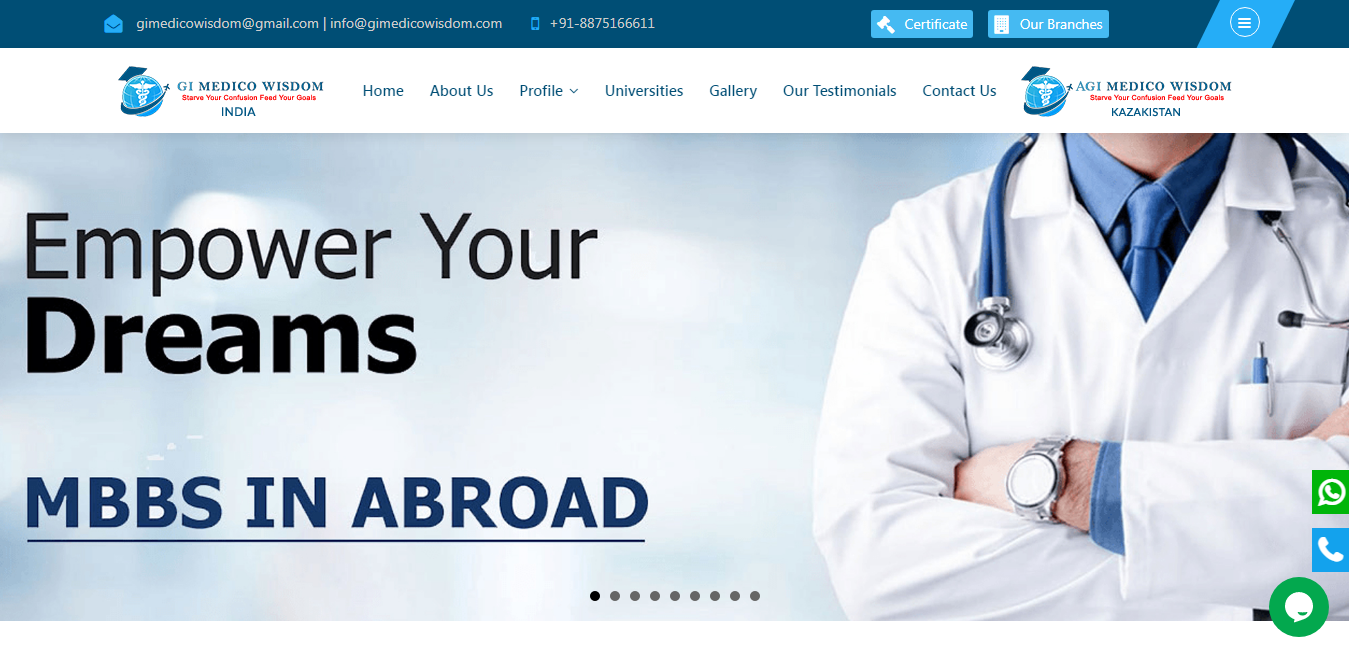This image prominently features a dark blue banner at the top, followed by a lighter blue section. In this lighter blue area, an open envelope icon appears alongside the text "GI Medico Wisdom." Below this, in a clear sequence, the email "GIMEDICOWISDOM@gmail.com" is displayed, followed by a vertical line leading to the text "info@gimedicowisdom.com." Adjacent to this, a light blue icon of a cell phone presents the contact number "+91-875-166611." On the right side of this section, in light blue squares, the headings "Our Certificate" and "Our Branches" are shown.

Descending further, a white banner spans the width of the image, featuring "GI Medico Wisdom India" followed by navigational options: Home, About Us, Profile, Universities, Gallery, Art, Testimonials, and Contact Us. At the bottom of the image, another banner carries the motivating slogan "Empower Your Dreams" in black text, alongside the phrase "MBBS in Abroad" in blue. The lower portion of the image visually captures a doctor with arms crossed, depicted from the neck to the waist.